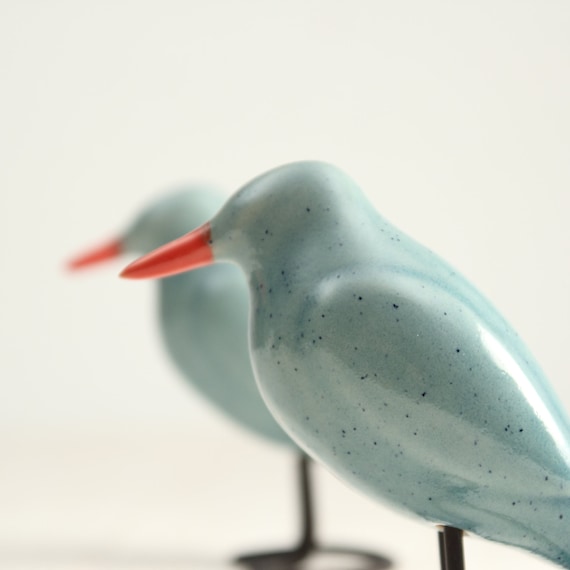The close-up image showcases two bird statues with smooth, lightly bluish-green bodies speckled with dark, nearly black dots. One bird is prominently in the foreground, revealing a vivid orange beak, while the other, nearly identical bird is faintly visible and heavily blurred in the background. Both birds are mounted on thin, black stands that extend into wide, flat bases, adding context to their positioning. The statues are devoid of intricate features like eyes, yet their distinct body shapes, upright poses, and slightly glossy feathers with bright white highlights catch the eye against the simple, light cream background. The scene is minimalist, accentuated by the reflection or shadow of the blurred bird in the background, emphasizing a somewhat ethereal symmetry.